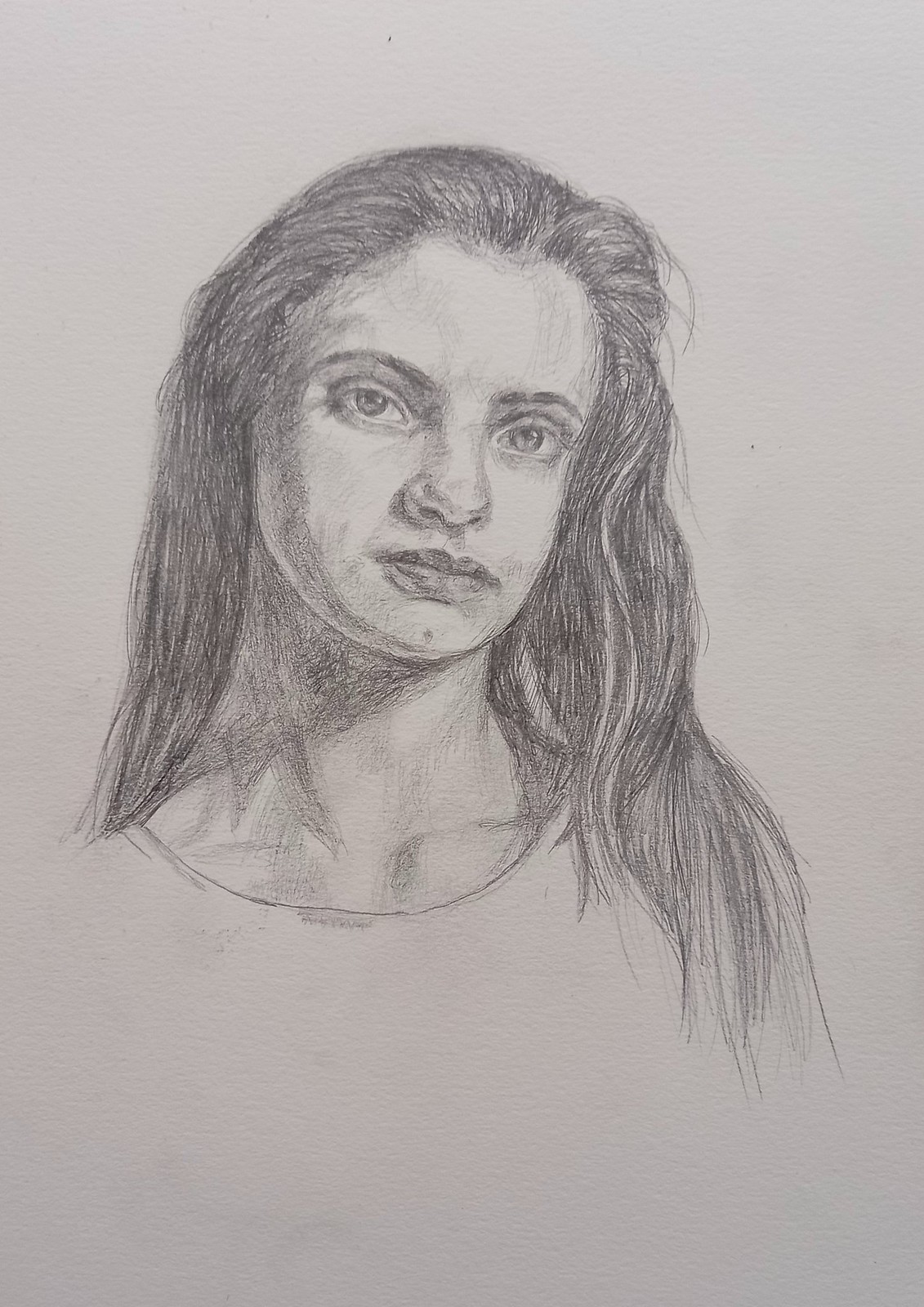This is a highly detailed pencil drawing of a woman on white paper, rendered entirely in black and white without any added colors. The portrait focuses closely on her face, showing her long, slightly wavy hair that extends past her shoulders, with most of it brushed back except for some strands on her left side (the right side from the viewer's perspective) that fall over her shoulder. Her facial features are defined by dark eyebrows, large eyes, a neutral expression with closed lips, and a distinctive mole at the center of her chin. The shading is particularly detailed on the left side of her neck, adding depth to the portrait. Only the upper portion of her torso is visible, delineated by the neckline of her top, with no other body parts such as arms or hands included in the image.